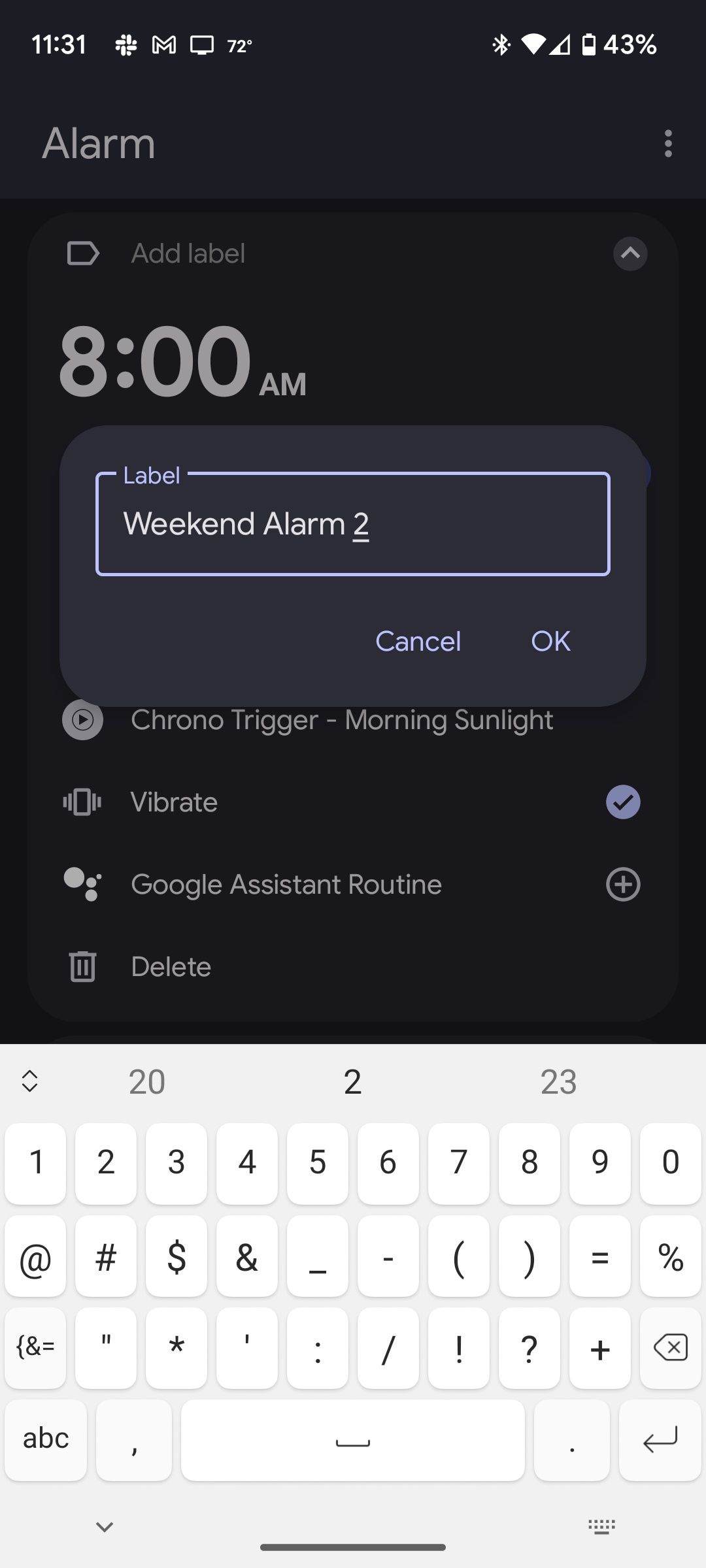A detailed screenshot of a cell phone interface with a black background. The status bar at the top features various icons: at the upper left, the time is displayed as 11:31. Nearby, there is a peculiar plus sign symbol, followed by the Google Mail icon, the Chromecast symbol, and a temperature reading of 72°F. The right side of the status bar shows additional icons: Bluetooth is enabled, Wi-Fi is fully connected, the cellular signal is at half strength, and the battery is at 43%.

Below the status bar, there's a gray notification area with gray text. On the left side of this area, the word "Alarm" is displayed, accompanied by three vertical dots. Below that, there's an open arrow pointing to the right, next to an "Add label" dropdown option. Further down, in gray text on the left side, the time is listed as 8:00 AM.

A pop-up window appears with a lighter gray background framed by a blue border. The word "Label" is highlighted in blue, with the text "Weekend Alarm 2" inside the box. The numeral "2" is underlined. At the bottom right of the pop-up, the options "Cancel" and "OK" are shown in gray text. Below these options, additional settings for the alarm include "Crawl trigger," "Morning sunlight," "Vibrate," "Google Assist Routine," and "Delete all," all in gray text.

At the bottom of the screen, the phone’s keyboard is visible, featuring white keys with black symbols. It is set to display numbers and special characters, showing the digits 1 through 9, 0, and symbols such as @, $, &, ?, and !.